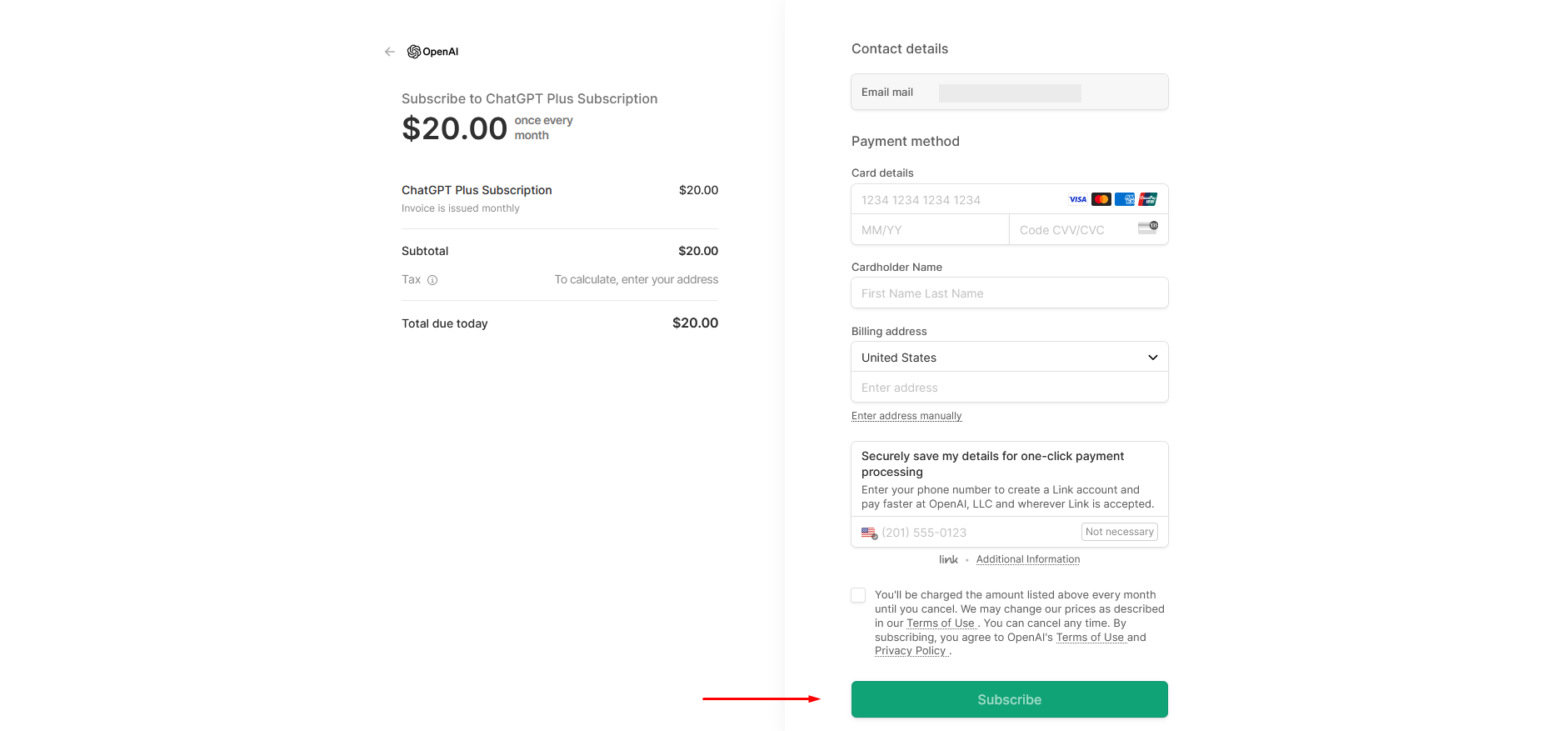The image is a detailed breakdown of a subscription payment page for ChatGPT Plus. 

On the left-hand side, the content is divided into structured sections. The first section prominently displays "ChatGPT Plus Subscription" in black, followed by the subscription cost of "$20.00" in gray. Below that, it states "Invoices issued monthly" in gray. Further down, there is a subtotal section that reads "$20.00" in black, with a note that tax is "To Be Calculated". The total amount due today is also listed as "$20.00" in black. A green horizontal line separates this from the other sections.

On the right-hand side, the caption in gray reads "Contact Details", accompanied by a green box containing blurred-out email details. Below this, the "Payment Method" section asks for card details, supporting Visa, MasterCard, and American Express. There are placeholders for the card number (formatted as 1234 1234 1234 1234), expiration date (MM/YY), CVV/CVC code, cardholder's first name and last name, and billing address, which defaults to the United States. There are options to "Enter Address Manually", "Securely Save My Details for One Click Payment", and a prompt to "Enter Your Phone Number to Create a Link".

At the bottom, a green box with a white "Subscribe" button is highlighted by a red arrow pointing towards it, indicating the final step to complete the subscription process.